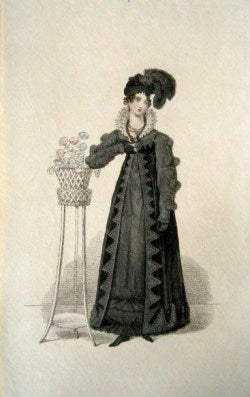This antique sepia-toned illustration depicts a pale woman with rosy cheeks, dressed in elaborate Regency or possibly Victorian-era attire, standing in a small white room. She wears a long, flowing black gown characterized by a high waist, lengthy sleeves, and layered garments that include a velvet coat, revealing an intricate design beneath. Her dress has a high collar that rises in the back and is lined with white fur or satin. Atop her head rests a black hat adorned with prominent feathers. The woman stands beside a tall, three-legged planter that reaches her waist. Her right arm gracefully bends with her hand resting on her chest, while her left arm hangs by her side, slightly stretching down. She gazes to her left, lending a subtle and poised elegance to her demeanor.